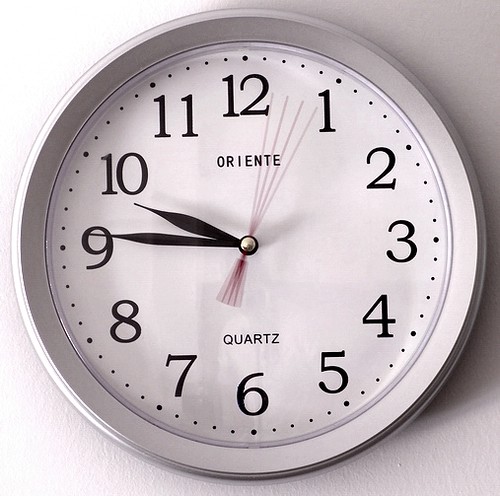This image features a small, round wall clock set against a wall with a textured white plaster or drywall finish. The clock itself boasts a white casing with a subtle lip extending slightly over the clock face. The face of the clock is bordered by a white ridge and adorned with black Arabic numerals, contrasting sharply against the white background. Small black dots mark the minute intervals between the hours. 

The clock's hands include a black hour hand, a black minute hand, and a red second hand. At the moment the photo was taken, the red second hand appears in motion, creating the illusion of four ghostly trails of red. Prominently displayed below the twelve o'clock position is the brand name "Oriente" in black lettering. Directly above the six o'clock position, the word "Quartz" is also inscribed in black, signifying the type of movement mechanism used in the clock.